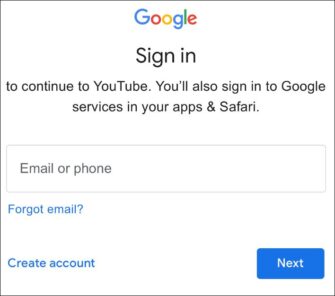A familiar scene plays out as you attempt to access YouTube using your Google account. The image features a stark all-white background with the iconic Google logo prominently displayed at the top center. The logo is composed of letters in various colors: the G in blue, the first O in red, the second O in yellow, the L in green, and the E in red. Below the logo, the black text "Sign in" invites users to proceed.

Underneath, the instructive message reads: "To continue to YouTube, you'll also sign in to Google services in your apps and Safari." There is a designated input field labeled "Email or phone" where users can enter their login credentials. Additionally, the phrase "Forgot email?" is highlighted in blue, offering a recovery option for those who can't recall their email address. 

At the bottom, the option "Create account" is also highlighted in blue, guiding new users through the account creation process. Beside this, a blue button with the word "Next" written in the center stands ready for the user to proceed with the login. The overall design is clean and minimalistic, with black lettering and blue highlights providing clear navigation cues against the white background.